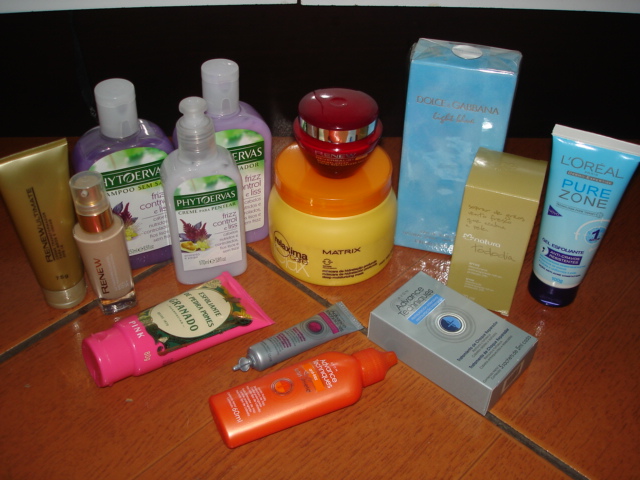On a surface tiled with large, light wood-grain tiles, a collection of assorted bottles, jars, boxes, and tubes is neatly arranged. In the foreground lies an orange bottle on its side, its white lettering blurred and unreadable. Just behind it, a small grayish-blue tube adds a touch of color, though its details remain indistinct. 

To the right of these, a grayish-blue box prominently displays the phrase "Advanced Techniques," though the rest of its writing is too blurry to discern. Amidst these items stands a large yellow jar with an orange lid boldly labeled "Matrix." 

Stacked atop this jar is a small maroon container with the word "Renew" clearly visible in silver lettering. Prominently featured in the center are three plastic bottles; the smallest one in the front is labeled "Phytoervas," and the two similar bottles behind it also bear the same brand name, "Phytoervas."

To the left, a beige bottle with vertical lettering spells out "Renew," standing tall beside an upside-down tube also marked "Renew." 

On the right side of the image, a tube labeled "L'Oreal Pure Zone" stands beside several indistinct boxes—one light blue, one light grayish-blue, and a tan box standing upright—though their inscriptions are illegible. The overall scene showcases a diverse array of personal care products meticulously arranged on a stylish, tiled surface.